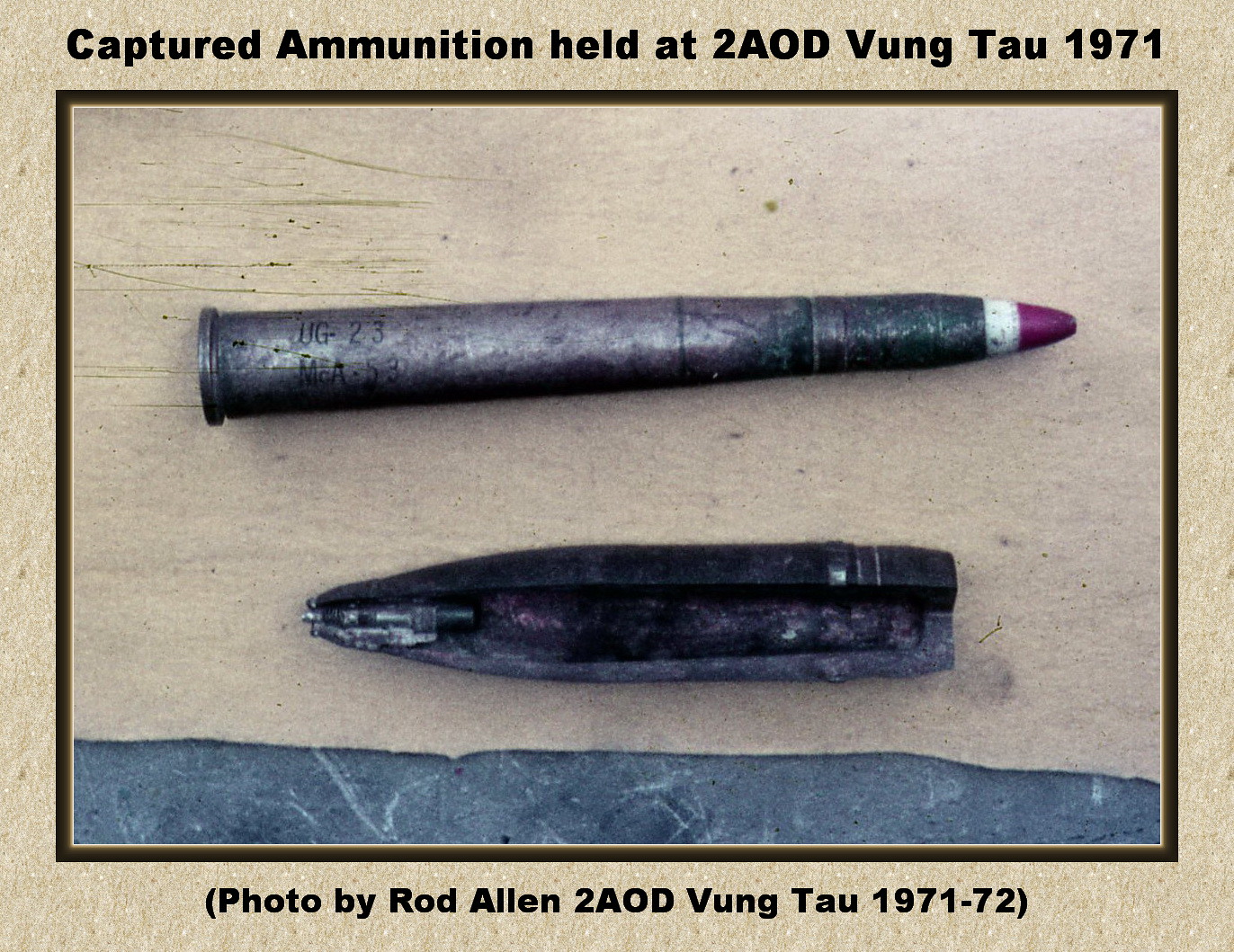This is a detailed photograph featuring two distinct pieces of captured ammunition displayed on what appears to be a wooden or fabric surface. Both pieces are annotated with their history and origin, specifically from 2AOD Vung Tau in 1971. The longer piece, resembling a crayon in shape, has a metallic silver base, a white body, and a purple, crayon-like tip. In contrast, the shorter piece is significantly wider and appears cracked, revealing its dark silvery-gray interior and pointed tip. Both pieces of ammunition bear the stamp "UG-23" and "MCA-53," emphasizing their precise identification. The photo is framed with a sandy, mottled yellow-brown border, accompanied by text both above and below the image. The top text reads, "Captured Ammunition Held at 2AOD Vung Tau, 1971," while the bottom credits Rod Allen as the photographer from 1971 to 1972. This well-focused photograph not only captures the intricate details of the ammunition but also provides significant historical context.